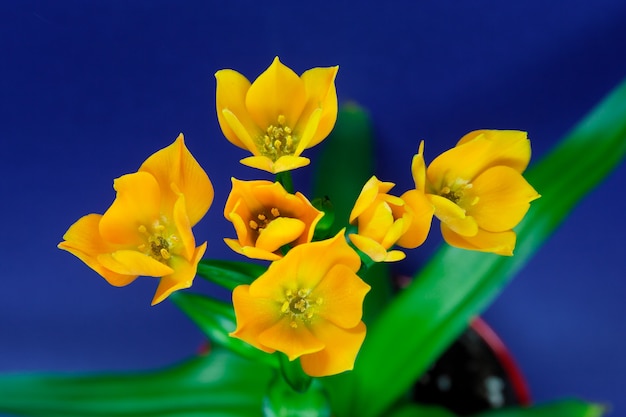The image captures a close-up of a vibrant plant with bright yellow flowers at the center. Each flower, boasting five or six pointed petals, reveals intricate details of tiny, light green stems tipped with yellow at the heart of the bloom. The plant is housed in a red pot, partially visible along with a glimpse of the rich soil at the bottom right corner. Surrounding the flowers are glossy, bright green leaves, with one prominent leaf stretching diagonally from the bottom middle to the upper right corner. Additional smaller leaves speckle the background, set against a serene blue backdrop. A noteworthy detail is that three flowers are fully open while another three remain partially closed, adding to the dynamic and lively composition of the photograph.